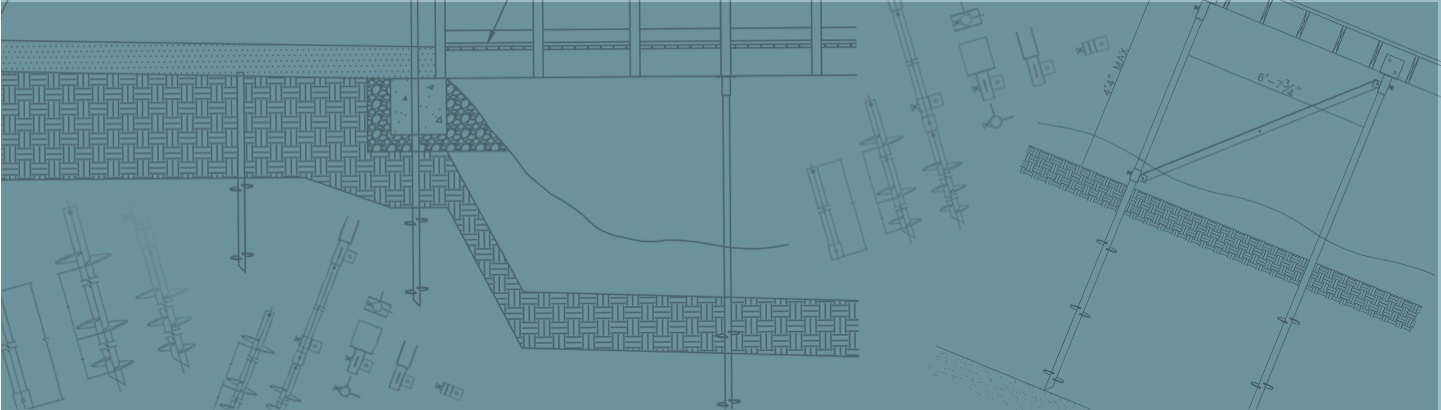The image is a blueprint-like digital design in landscape orientation, featuring a narrow, rectangle shape with a predominant bluish-gray or teal color background. Overlaid in gray, the design resembles an architectural or engineering sketch, filled with numerous intricate details. This includes sketches and diagrams of interconnected poles forming a thatchwork, and multiple drill-like structures scattered across both the left and right sides. There's a depiction of tracks of land segmented by fences and levels that suggest a basement-like structure with cross-hatching and poles. A river-like line runs horizontally from almost left to right, intersecting the layout. Towards the right side, there's a large braced mechanism with additional drill elements attached. The only discernible text on the image is a few equations on the right side, although it's generally difficult to read.